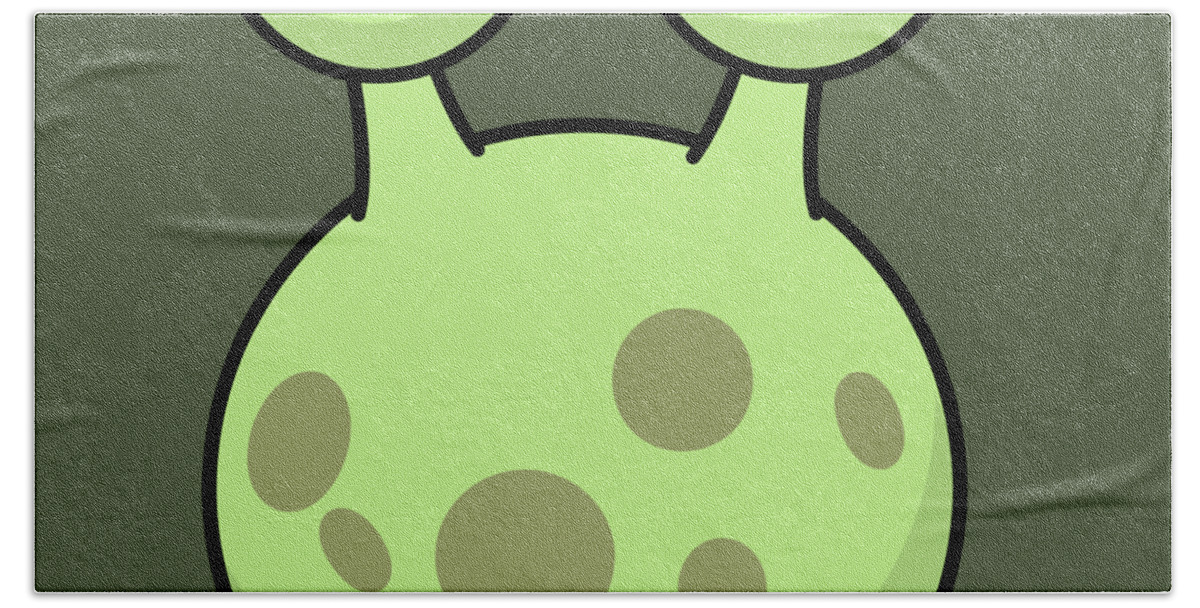The image is a detailed illustration of a lime green, cartoonish alien head set against a darkish olive green background. The alien head is outlined in black and features two antenna-like stalks protruding from its top, both of which terminate abruptly where they begin to form another circle, as if cut off. The head itself is decorated with six distinct spots, varying in size and shape, some being circular and others oblong ovals, filled with a dark green-grey color. The arrangement of these spots includes positions such as center-right, far-right, bottom-right, bottom-left, far-bottom-left, and bottom-left, adding to the whimsical and peculiar appearance of this alien creature. The overall design has a playful, yet mysterious aesthetic, reminiscent of a close-up cartoon depiction often seen in posters or themed illustrations.